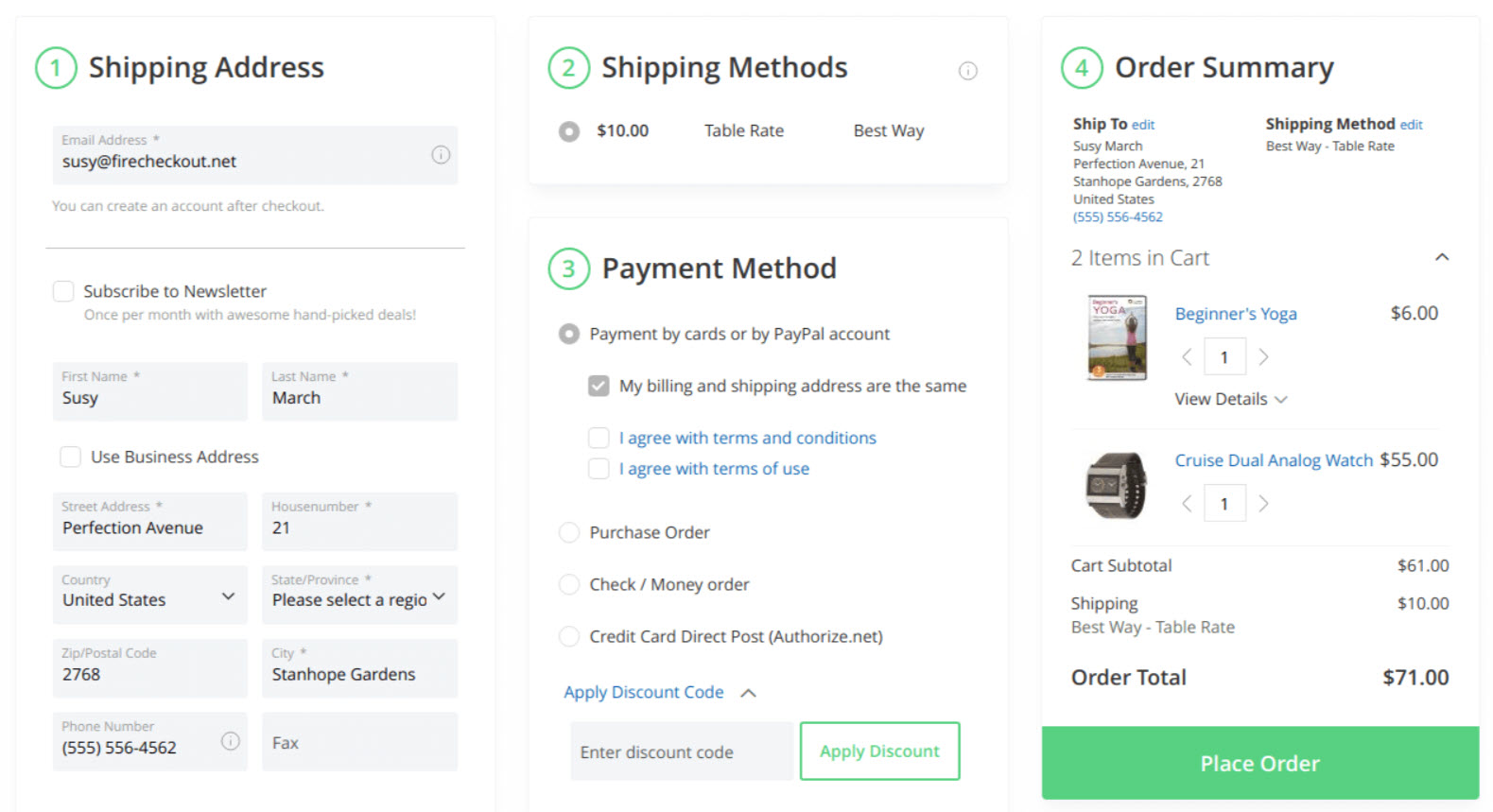On this image, an order form is prominently displayed, divided into four main steps, each marked by numerals 1 through 4 in green. 

**Step 1: Shipping Address**
- Positioned at the top-left corner.
- Fields for Email Address, First Name, Last Name, Street Address, House Number, Country, State, Zip Code, City, Fax, and Phone Number.
- Example Email: sassy@firecheckouts.net.
- Option to create an account post-checkout.
- Checkbox to subscribe to the newsletter.
- Checkbox to use a business address.

**Step 2: Shipping Method**
- Available method: $10 Table Rate - Best Way.

**Step 3: Payment Method**
- Options to pay by card or PayPal.
- Checkbox to indicate: "My billing and shipping address are the same."
- Other payment methods include Purchase Order, Check, Money Order, Credit Card Post, and Authorized.net.
- Discount space with a green "Apply Discount" button.
- Agreement checkboxes in green and blue text: "I agree with terms and conditions" and "I agree with terms of use".

**Step 4: Order Summary**
- Shipping address re-iterated.
- Confirmed shipping method from Step 2.
- Items in the cart: Beginner's Yoga priced at $6 and Cruise Dual Analog Watch priced at $55.
- Cart Subtotal: $61
- Shipping: $10
- Order Total: $71.
- Prominent green "Place Order" button located at the bottom-right.

The form is structured for clarity, with designated fields and options to ensure all necessary purchase details are collected efficiently. The green and blue colors provide visual cues for important actions and acknowledgments.